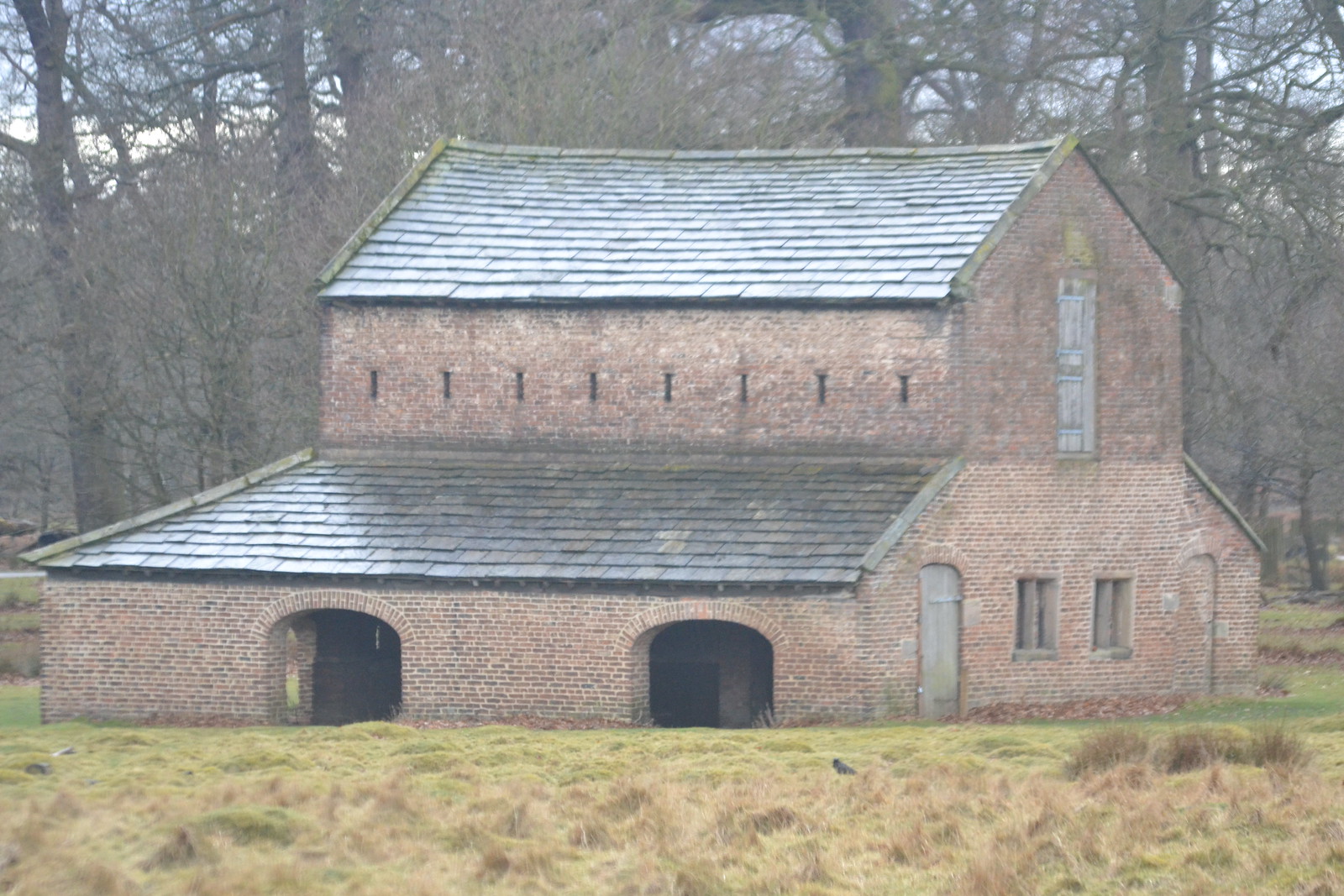This color photograph, taken outdoors during the daytime in a very rural setting, captures a picturesque scene reminiscent of the British Highlands. The foreground features an expansive, unmanicured field with long grasses covering gentle, undulating hills. A few bushes dot the landscape, enhancing the rustic charm. 

In the background, trees devoid of leaves frame the scene against a sky scattered with clouds, suggesting the photograph was taken in late fall or winter. 

Dominating the mid-ground is a two-story brick building with a black roof. The building, viewed from its longer side, reveals two large arching entryways on the first story. It also features about eight or nine small slot windows, contributing to its intriguing architecture. The building's base is wider than its top, with sides that taper diagonally. 

On the visible side, there are several doors and windows, including a curious door on the second story that leads to nowhere, hinting at an erstwhile use or design quirk. This door, evidently, if opened, would lead straight to the ground below. The structure, with its distinctive shape and elements, evokes the look of a small arcade, adding to the scene’s historical and cultural texture.